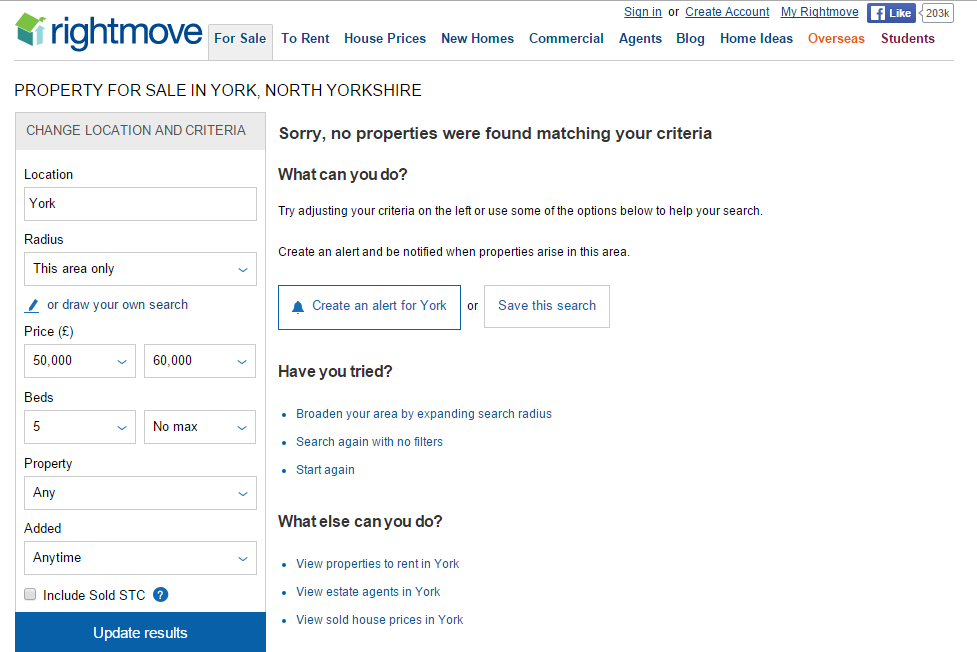The image is a screenshot of a real estate website with an immaculate and user-friendly design, primarily against a white background with distinctive borders. The photo is landscape-oriented and showcases the website’s top navigation area with a thin black border at the top of the screen and a gray border underneath, creating a well-defined header. 

At the top-left corner, there is a logo featuring an image of a house colored in green, blue, white, and light blue hues, accompanied by the text "Right Move" to its right. Adjacent to the logo, there are several clickable tabs including "For Sale," "To Rent," "House Prices," "New Homes," "Commercial," "Agent," "Blog," "Home Idea," "Overseas," and "Students." The “For Sale” tab is highlighted in gray with a box around it. The “Overseas” tab is marked in orange, while the “Students” tab appears in a maroon font. 

Above the tabs, there are additional links for user navigation: "Sign In," "Create Account," "My Right Move," and a Facebook Like button. 

Just below the border, a prominent header reads "Property for sale in York, North Yorkshire." On the left side, there's a vertical box labeled “Change location and criteria,” which includes fields for "Location and Radius," an option to "Draw your own search," price in Euros, selectable "Number of Beds" with minimum and maximum filters, and an option for "Property Added."

To the right of this box, a message informs the user that "No properties were found matching your criteria." It suggests adjusting the search criteria on the left or utilizing other options below. It advises users to "Create and add an alert to be notified when properties arise," with an easy-to-find button to create or save their search criteria.

This detailed and organized layout demonstrates the site’s commitment to user experience, providing a clear and accessible interface for navigating real estate options.